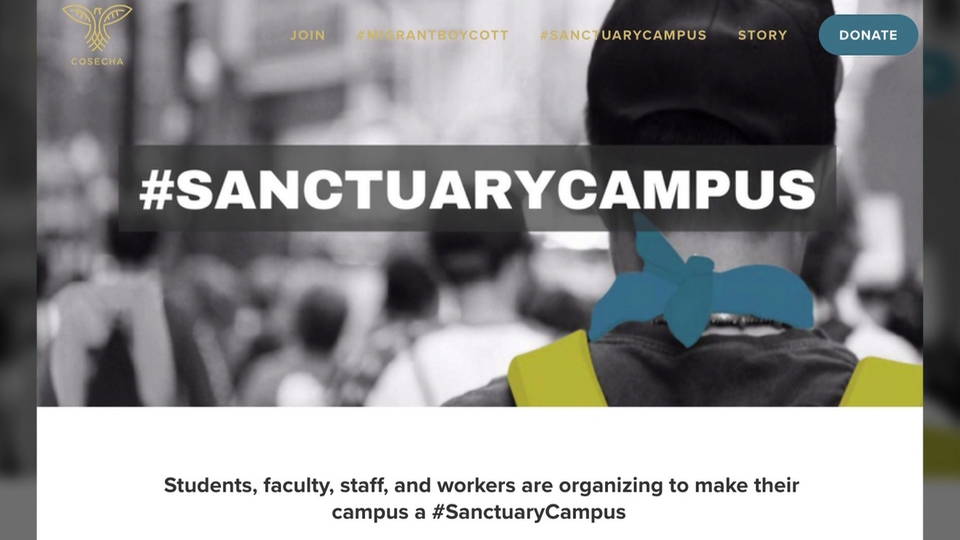This screenshot appears to capture a section of a website with a distinct layout and visual elements. In the upper left corner, there is a stylized bird logo next to the word "C-O-S-E-C-H-A," both rendered in a bright yellow font. The main image on the website depicts a crowd of people walking away from the camera, with one individual on the right side prominently featuring the strap of a yellow backpack. At the top of the website, the navigation menu includes the word "Join" and phrases such as "Sanctuary Campus Story." There is also a partially obscured word related to a "boycott." Additionally, the center of the image features the hashtag "#SanctuaryCampus."